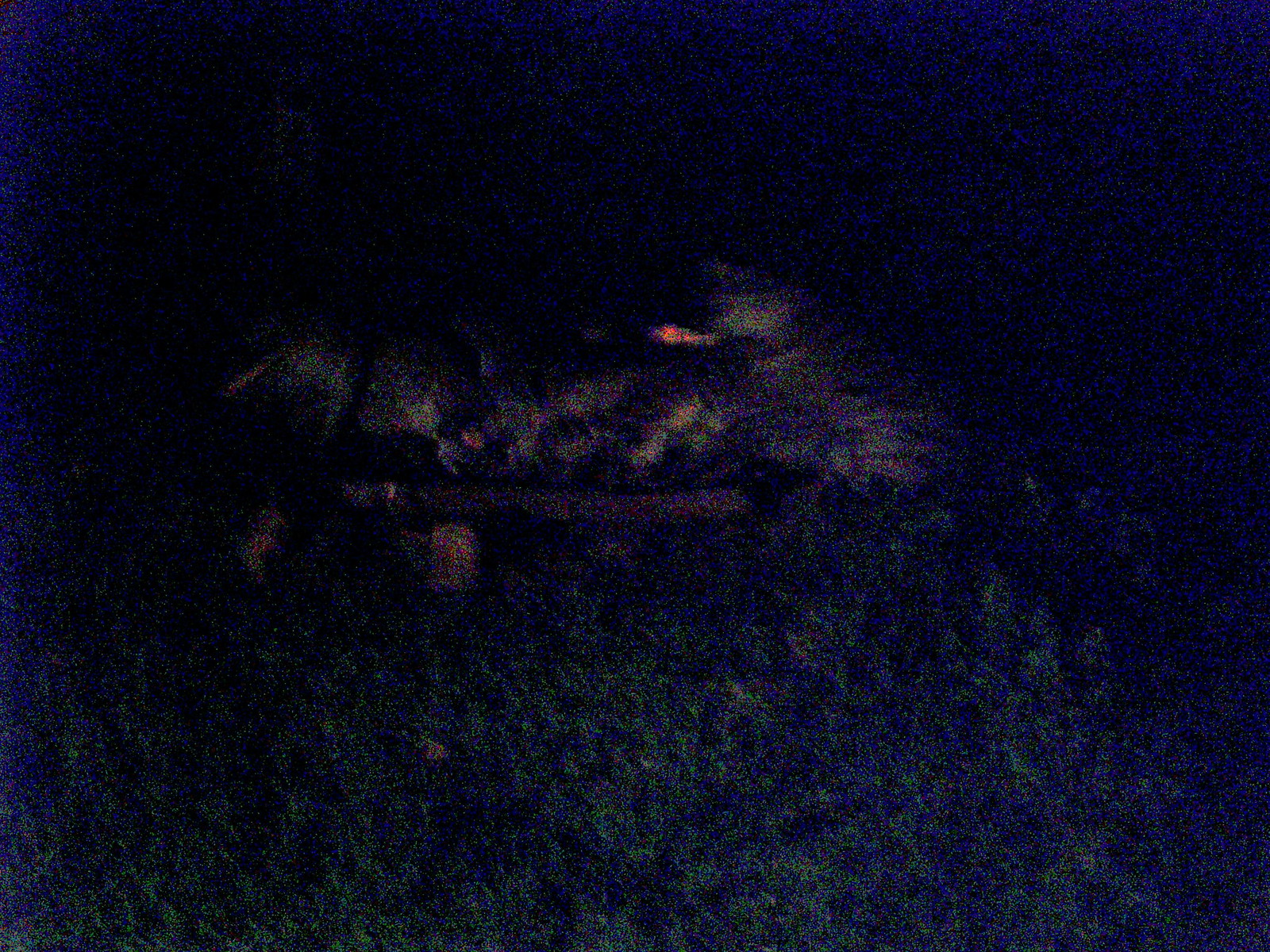The image presents a very blurry scene of a field adorned with purple flowers. Nestled amidst the blossoms is what appears to be an animal, distinctive with its long hair and visible red mouth. The creature, lying on its side with its head turned backward, is surrounded by vibrant colors, adding a sense of depth despite the image's lack of clarity. Nearby, a piece of wood is discernible, contributing to the rustic ambiance of the setting. Although the indistinctness of the photograph complicates the details, the presumed animal seems to have paws, providing a clue to its identity in this picturesque yet enigmatic tableau.